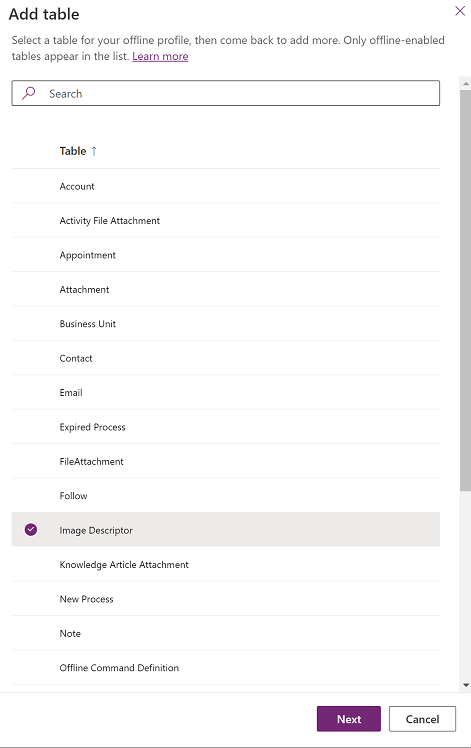In the top left of the image, the text "Add Table" is prominently displayed in black. Directly below this, a series of instructions reads, "Select the table for your offline profile, then come back to add more. Only offline enabled tables appear on the list." The phrase "Learn more" is highlighted in purple and underlined. Beneath these instructions, a rectangular search box stretches across the image, featuring the word "Search" in purple with a magnifying glass icon to its left.

Descending from this search box is an alphabetically ordered list of table names, beginning with the bolded black title "Table." The listed items include: "Account," "Activity File Attachment," "Appointment," "Attachment," "Business Unit," "Contact," "Email," "Expired Process," "File Attachment," "Follow," and "Image Descriptor." Notably, "Image Descriptor" has a white checkmark enclosed in a purple circle next to it, standing out against a gray background, in contrast to the white background of the other items. The list continues with "Knowledge Article Attachment," "New Process," "Note," and "Offline Command Definition."